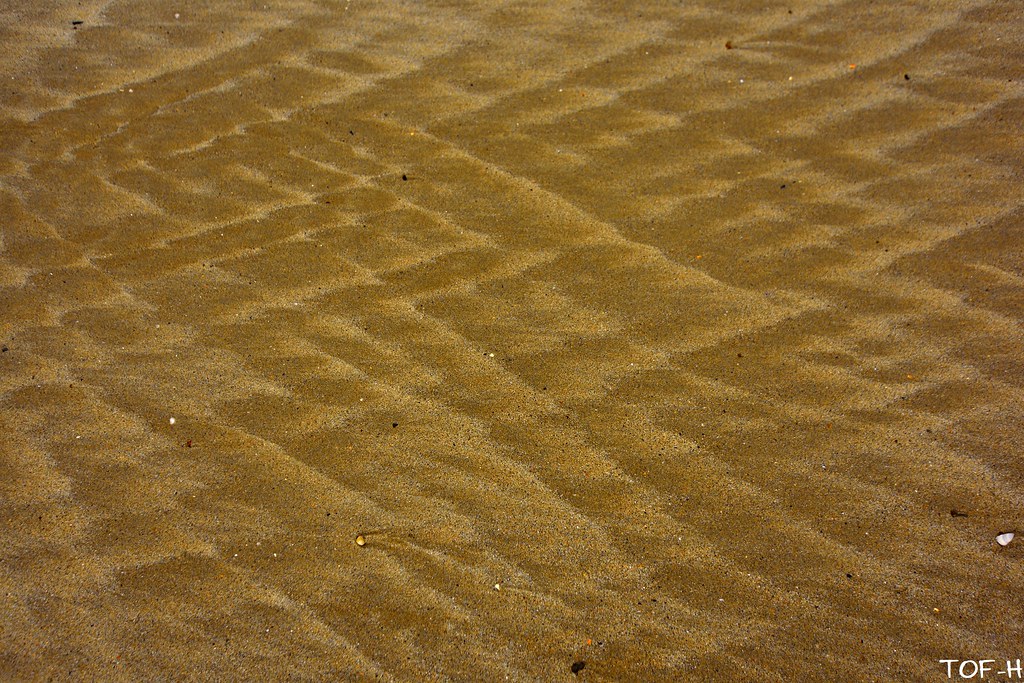This photograph captures a section of a beach, revealing intricate ripple patterns in the wet sand created by the ebb and flow of the tides. The main color palette consists of various shades of brown, ranging from light beige to deeper honey tones. Scattered across the sand are tiny rocks and pebbles in shades of white, black, beige, and brown, adding texture and depth to the scene. Notably, a larger white rock is visible near the bottom right corner, while smaller black rocks can be found towards the middle and lower parts of the image. The photograph, taken during daytime, has a somewhat indistinct and understated appearance. It measures approximately six by six and features the initials "TOF-H" in small white text at the bottom left, likely marking the photographer's signature or possibly the image number.